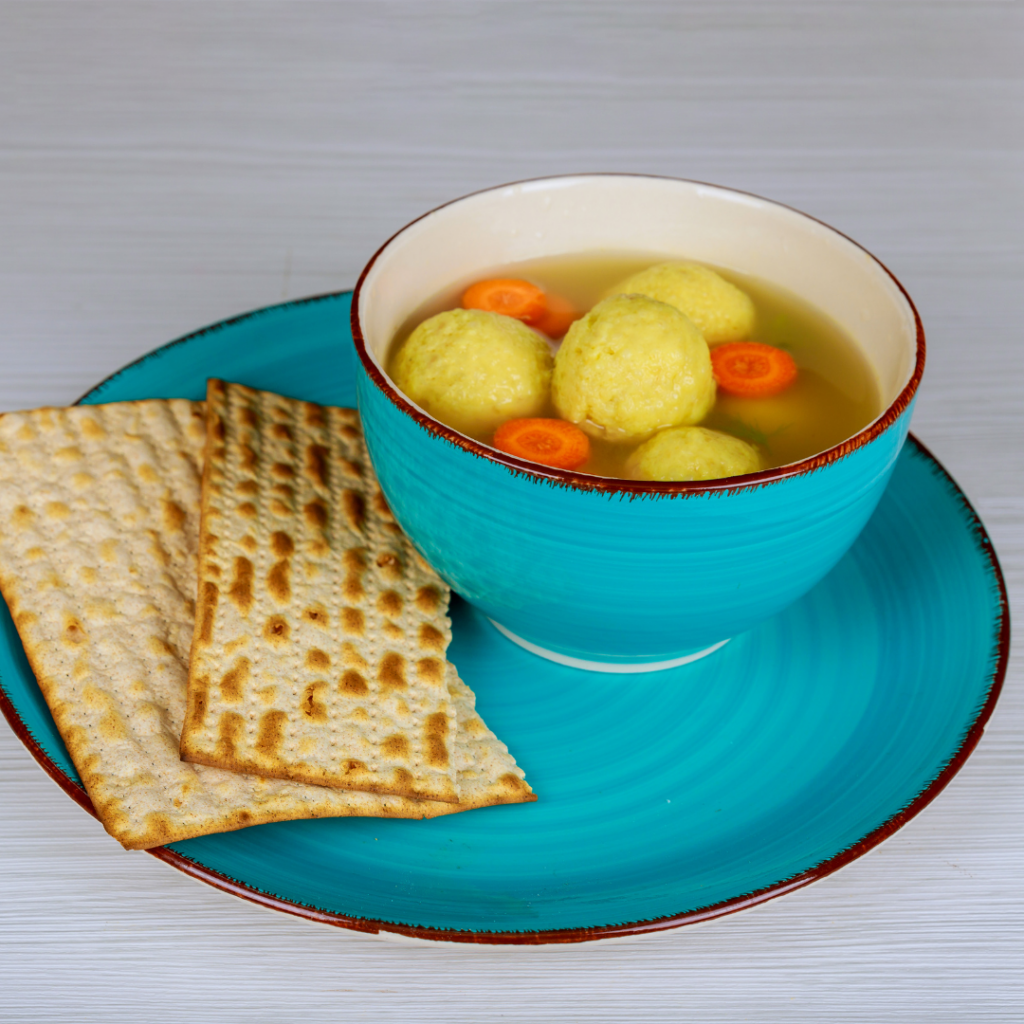This color photograph features a meticulously arranged serving of matzo ball soup and matzo crackers set against a white painted wooden background. The ceramic bowl and plate share a turquoise blue color scheme, contributing to a cohesive and visually appealing presentation. The bowl, stacked on the plate, contains four large, yellow matzo balls immersed in a yellowish, possibly chicken or vegetable broth, which has a slightly muddy, dark golden hue. Bright orange carrot slices add a pop of color to the soup. Next to the bowl, within the plate, rests a matzo cracker broken in two, showcasing a light brown and slightly toasted finish. The composition is clean and professionally presented, highlighting the traditional Jewish dish often enjoyed during Passover.